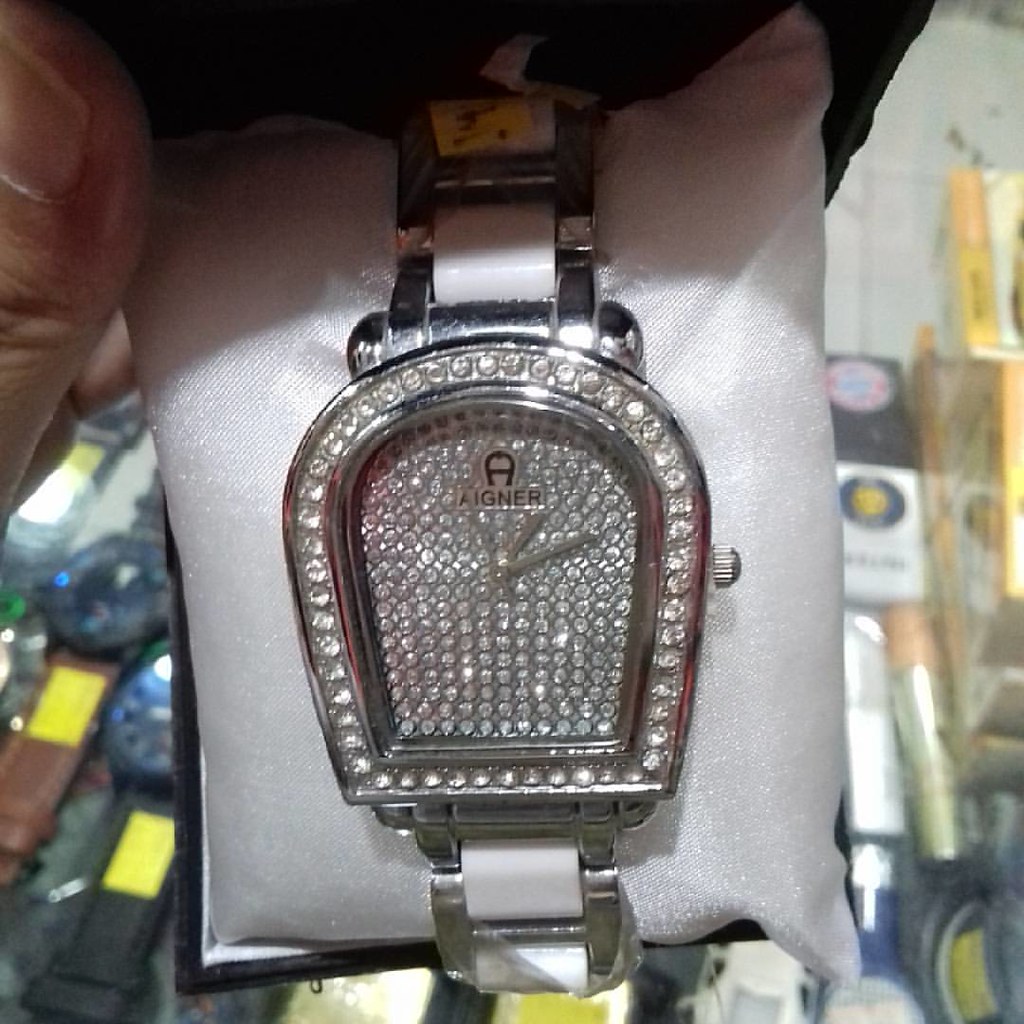In the background, a display case showcases an array of watches adorned with yellow price tags. Notably, one watch features black straps with a traditional clock face, displayed next to another watch with a similar design. Another watch, sporting brown straps, accentuates the collection. However, the centerpiece is a dazzling timepiece with metal straps, encrusted with diamonds encircling the clock face. Additional diamonds embellish the interior of the watch face, where two metal hands delineate the time — a long hand for minutes and a shorter one for hours. An intriguing detail is an 'A' symbol, designed as a rounded capital letter, accompanied by the brand name 'Anye' printed in block letters beneath it.